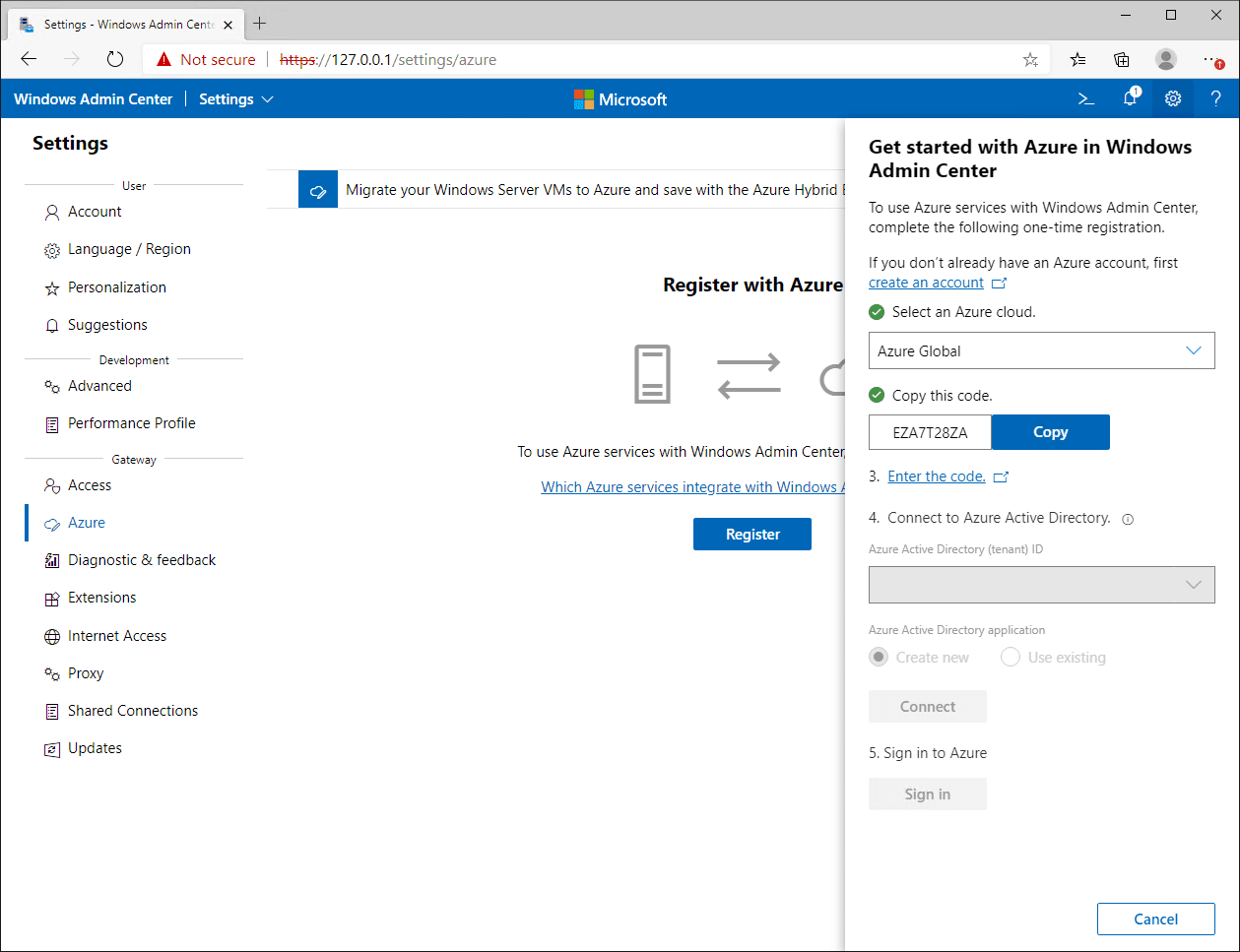This image is a detailed screenshot of the Windows Admin Center settings page, specifically the "Register with Azure" section. The URL in the top address bar is "http://127.0.0.1/settings/azure", which is marked as "Not Secure" with a red typeset and a red triangle icon. The "HTTPS" protocol is crossed out, indicating the absence of a secure connection.

The main settings page has a sidebar on the left-hand side, displaying various settings categories which include: Account, Language & Region, Personalization, Suggestions, and Development. Under the Development category, several sub-options are listed: Advanced Performance Profile, Gateway, Access, Azure, Diagnostic & Feedback, Extensions, Internet Access, Proxy, Shared Connections, and Updates. The "Azure" option is highlighted in blue, indicating it is the current selection.

On the right-hand side of the image, there is a vertical column providing instructions on integrating Azure with the Windows Admin Center. This column includes information on how to copy the necessary code for this integration.

The page features a clean, organized layout with a color scheme primarily consisting of white, blue, and green. The Microsoft logo, displayed in its traditional colors of green, red, blue, and yellow, adds a touch of branding to the page.